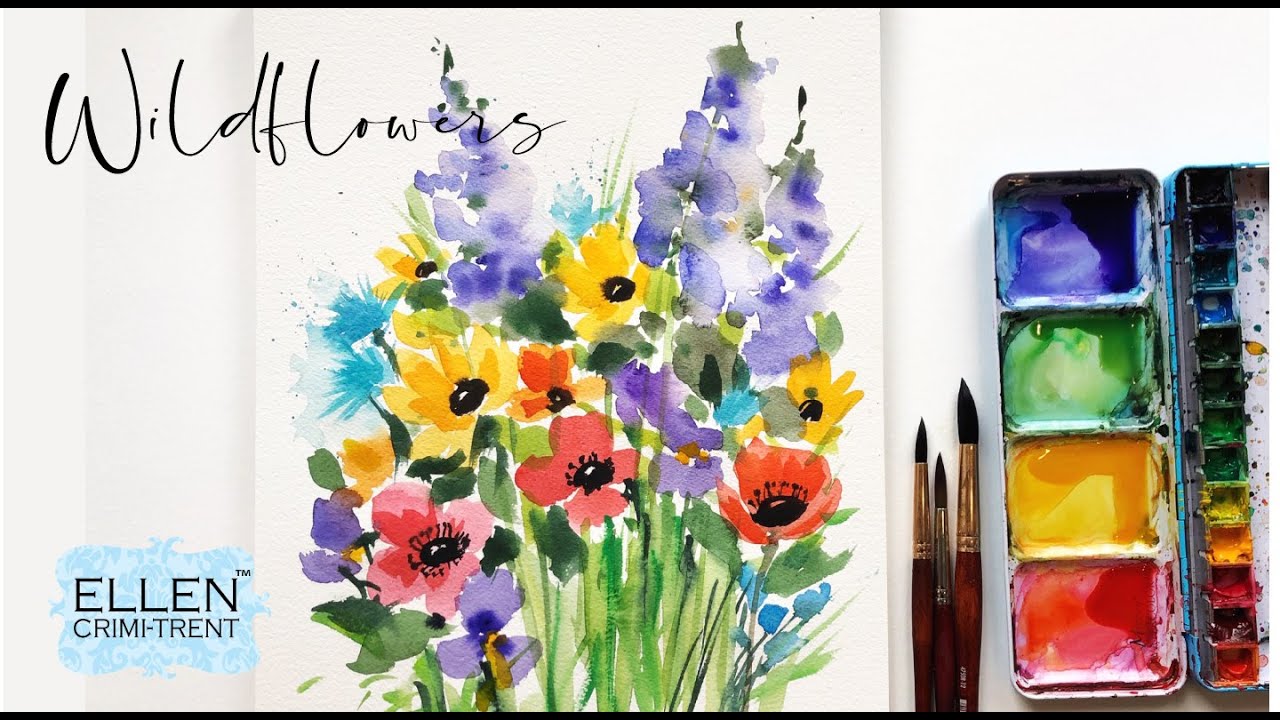This image is a book cover with a landscape rectangular layout on a white background. At the center is an elegant painting of a wildflower bouquet in muted pastel shades of rose, violet, yellow, and blue. The wildflowers, some with dark centers, are complemented by green foliage. At the top left, in a cursive font, it reads "Wildflowers." In the bottom left corner, over a patch of blue watercolor, is the author's name, Ellen Crimi-Trent, written in black letters. On the right-hand side of the image is a sophisticated watercolor paint tray, featuring primary colors of violet, green, yellow, and red, with additional smaller compartments holding various shades of these colors. Adjacent to the paint tray are three paintbrushes with brown handles and gold ferrules.